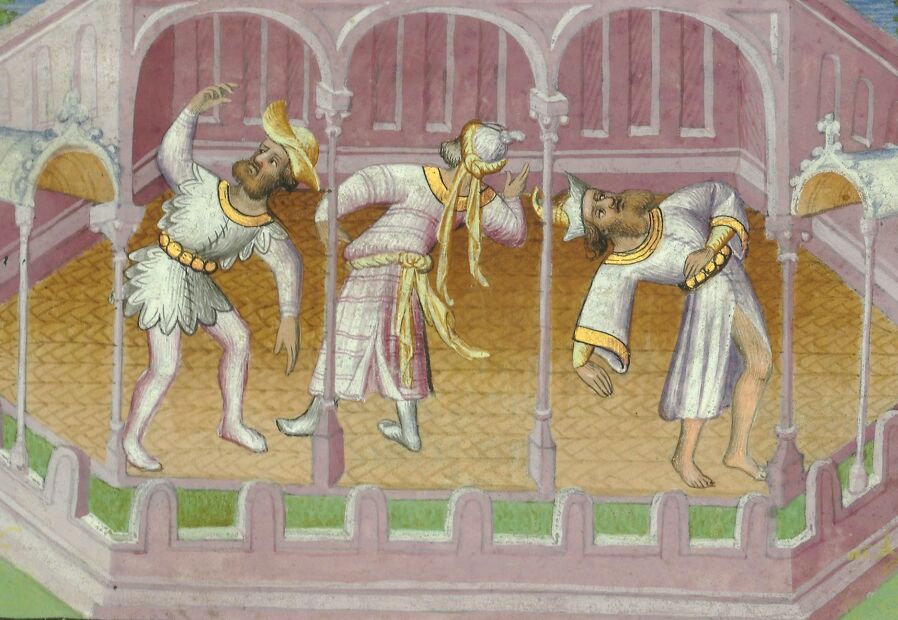The image is a full-color, horizontally rectangular painting that appears to represent a scene from the Middle Ages. It features three men dancing in an open, arch-filled room with a pink back wall and a white archway in the center upper right. The floor they are dancing on is yellow with woven V-shaped patterns running horizontally. The bottom of the image shows a pink wall that acts as a low border.

The men are adorned in medieval attire. The man on the left is dressed in a short tunic with a yellow hat that resembles a cowboy hat. He has pink stockings and a gold belt, and his posture shows him bent at the knees with his left arm raised above his head, looking up, and his right arm hanging down.

The man in the middle is facing away from the viewer, dressed in a long pink and white tunic with white boots. He is leaning back with his right hand near his head and his left hand by his waist. His legs are spread apart, contributing to the dynamic posture of the dance.

The man on the right wears a long white tunic. He is leaning back dramatically, his left arm bent near his waist, and his right arm thrown back behind him. His garments and positioning suggest an active motion, contributing to the overall sense of movement within the painting.

This detailed depiction of the trio captures their intricate dance moves, highlighting the vibrant and evocative nature of medieval artistry.